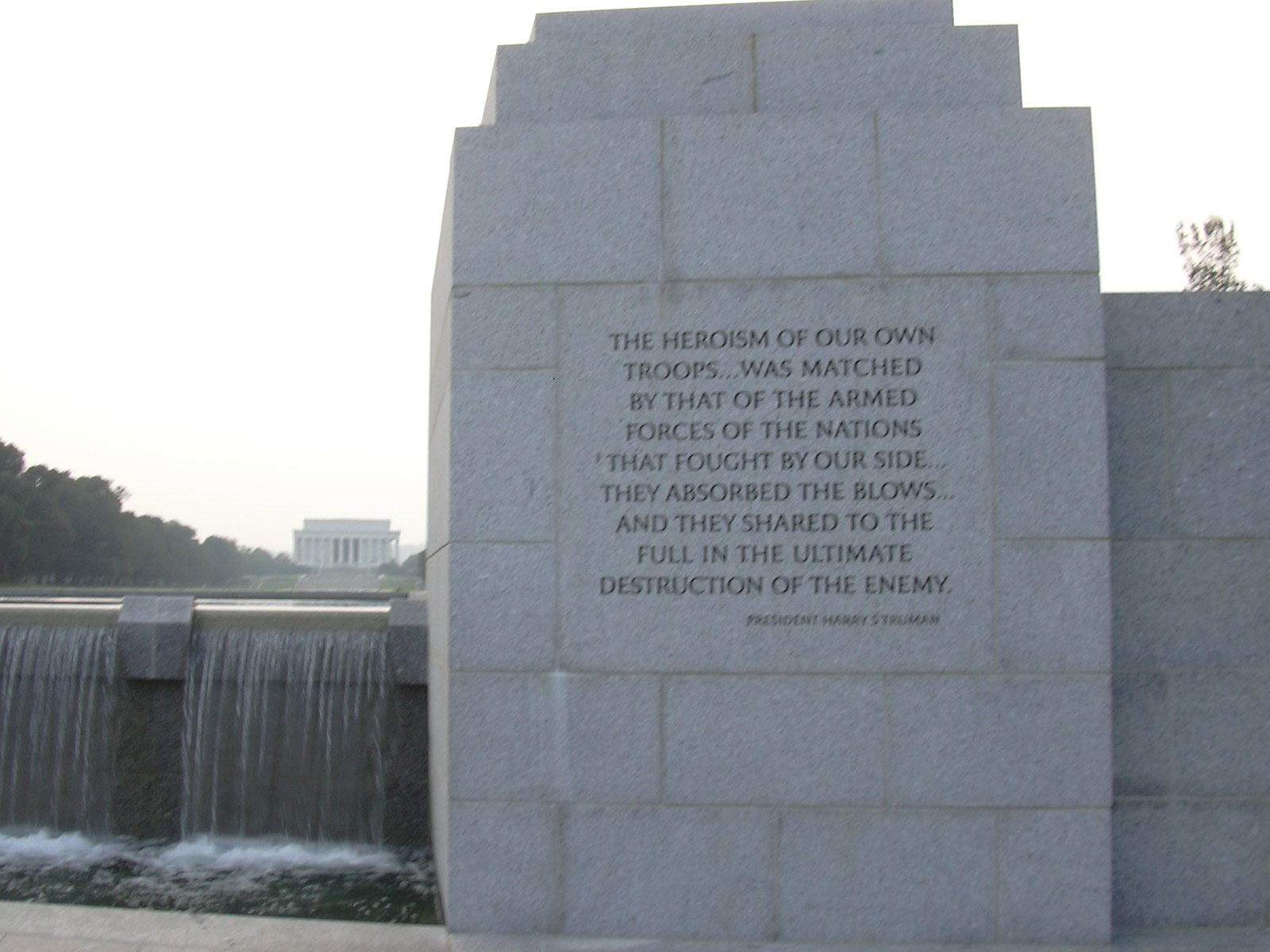This is a large, square photograph capturing a World War II memorial. The focal point is a tall stone wall inscribed with a tribute: "The heroism of our own troops... was matched by that of the armed forces of the nations that fought by our side... They absorbed the blows... and they shared to the full in the ultimate destruction of the enemy." Beneath this, smaller text attributes the quote to President Harry S. Truman. The upper parts of the image are dominated by a white sky, indicating an overcast day.

To the left of the memorial wall, a cascading waterfall flows, suggesting it is part of a larger commemorative setting. In the background, there is a notable political building, which resembles the Lincoln Memorial, further encircled by a dense cluster of trees on the far left side. The combination of natural and architectural elements, alongside the memorial's profound inscription, creates a somber and reflective scene.